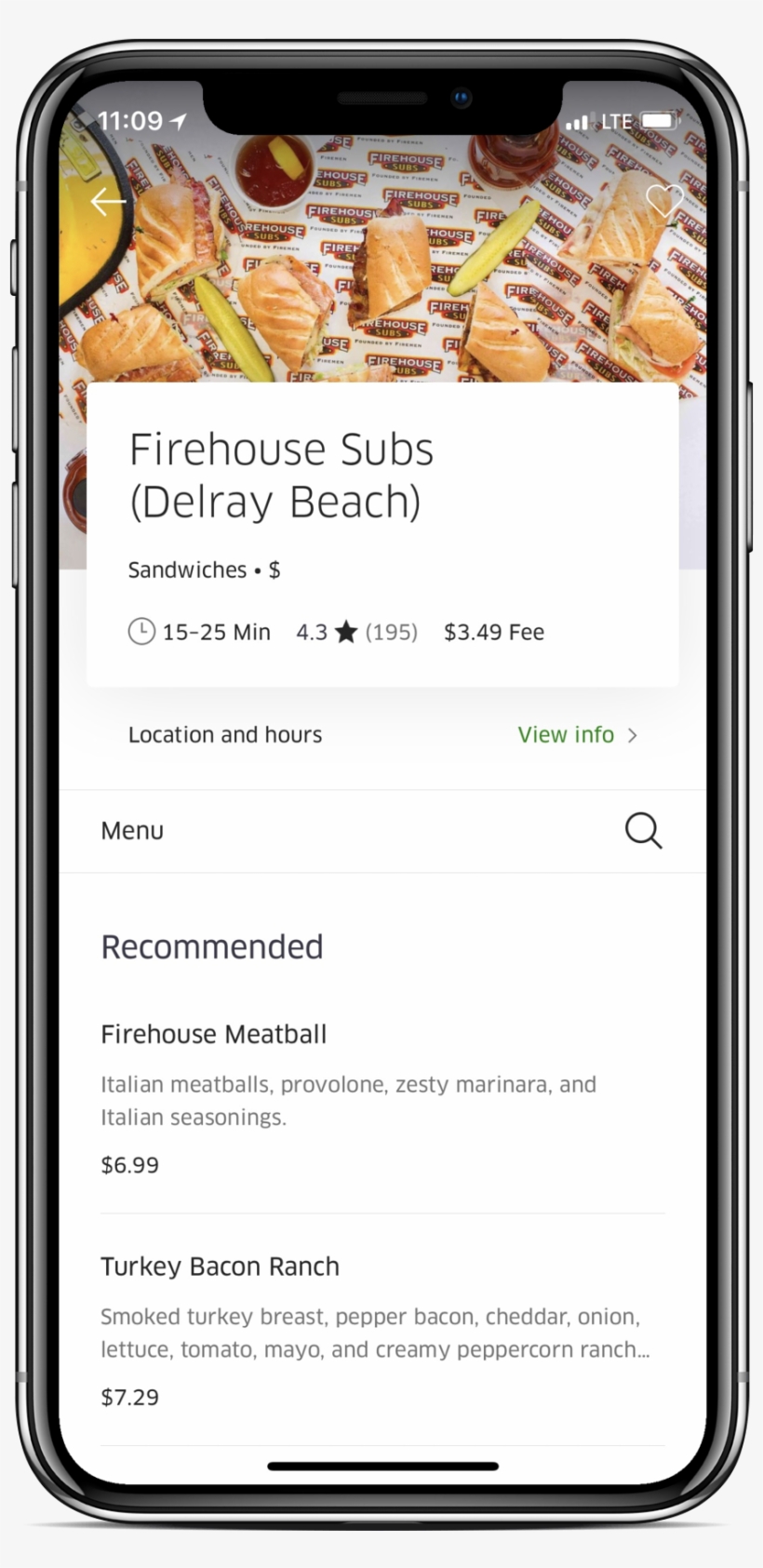This is an image of a mobile phone screen displaying details of a restaurant entry on a food delivery app. At the upper left corner of the screen, the time is shown as 11:09, while at the upper right corner, there is an LTE signal indicator with three bars for connectivity strength and a battery power icon. 

The entry featured is for "Firehouse Subs," located in Delray Beach, which is indicated in parentheses below the store name. The background of the entry is decorated with the Firehouse Subs’ signature graphic. The entry summary showcases various details: the restaurant serves Sandwiches and is categorized by a single dollar sign ($), indicating its pricing level. The estimated delivery time ranges from 15 to 25 minutes.

The restaurant has a rating of 4.3 stars and mentions a delivery fee structure with $1.95 displayed in parentheses alongside the primary fee of $3.49. Below these details, there are clickable options such as "Location and Hours," "View Info," and "Menu," with a magnifying glass icon next to "Menu," implying a search function.

The recommended items from the menu are highlighted with detailed descriptions and pricing. One option is the "Firehouse Meatball" sandwich, which contains Italian Meatballs, Provolone, Zesty Marinara, and Italian Seasoning, priced at $6.99. Another recommendation is the "Turkey Bacon Ranch" sandwich, composed of Smoked Turkey Breast, Pepper Bacon, Cheddar, Onion, Lettuce, Tomato, Mayo, and Creamy Peppercorn Ranch, costing $7.29.